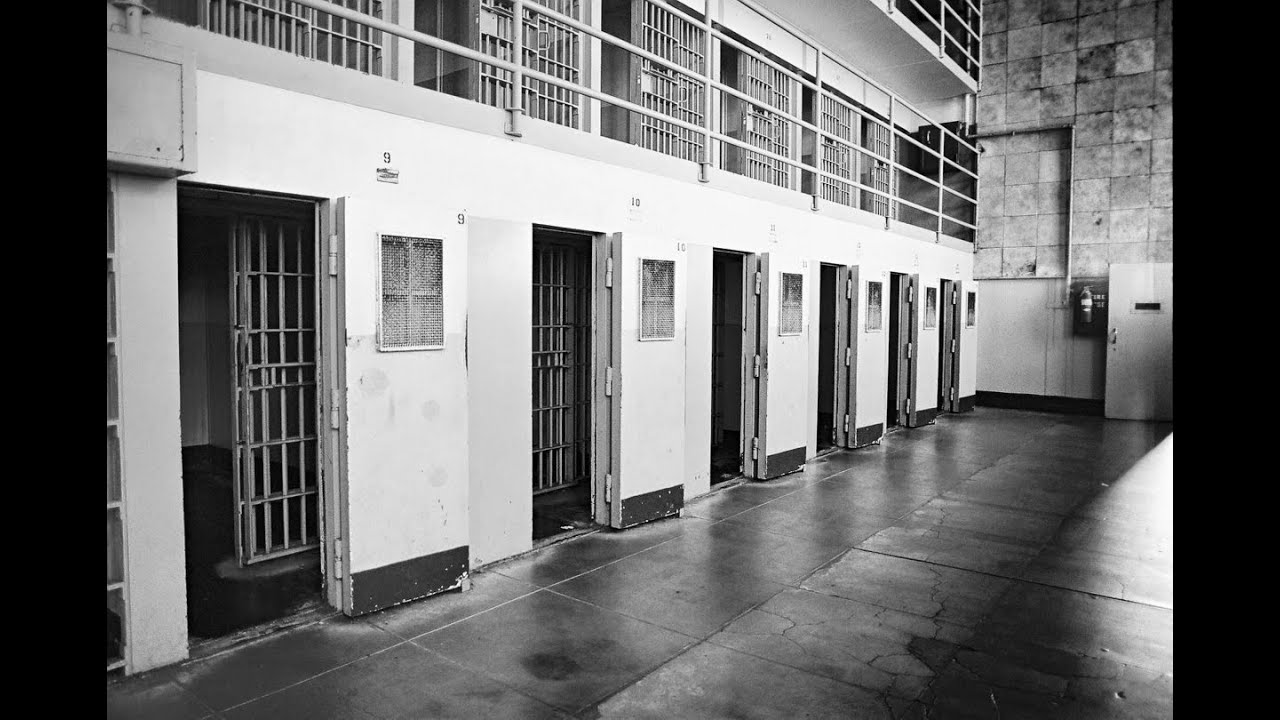This black and white photograph depicts the interior of an old jail, showcasing a stark, desolate environment. The scene captures a hallway with a cement floor and features two levels of open jail cells, with a glimpse of a partial third level. Each cell is barred, and several doors are visibly open. The numbered cells, notably 9 and 10 on the bottom left, accentuate the institution's organizational rigidity. The walls are constructed from rock and tiles, contributing to the austere atmosphere. A guardrail on the upper level prevents falls, adding a measure of safety to the spartan environment. The absence of prisoners coupled with the drab color palette—shades of gray, black, and dull white—emphasizes the bleakness. The only notable item is a fire extinguisher encased on the wall, hinting at basic safety measures in an otherwise grim setting.